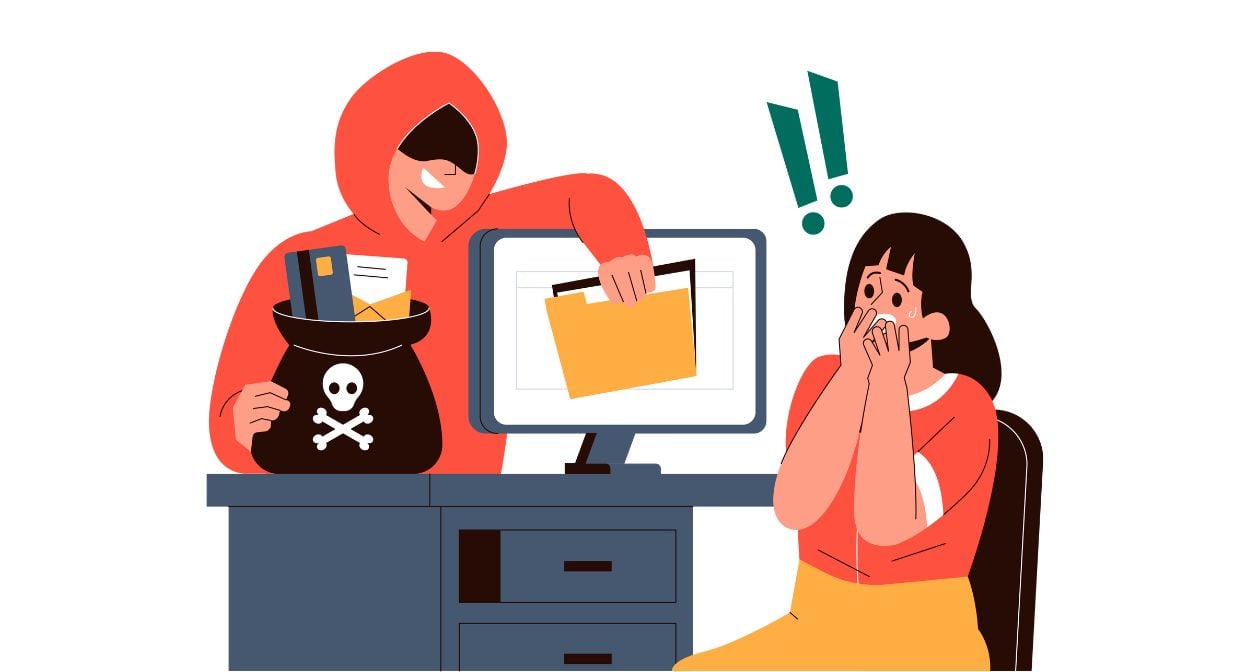This detailed cartoon image on a white background showcases a dramatic scene. A woman, dressed in a red shirt with white trim and yellow bottoms, sits at a blue desk in a brown office chair. The desk, featuring two drawers with one slightly open, supports a matching blue computer monitor displaying a white screen. The woman is visibly alarmed, with both hands clasped around her mouth and two green exclamation points hovering above her head, indicating her panic.

Behind the desk stands a man in an orange hoodie with his face masked, epitomizing a sinister hacker. He holds a black bag marked with a white skull and crossbones, containing credit cards and papers. This hacker reaches across the desk and through the computer monitor, seemingly inserting harmful files or extracting sensitive information, signifying an act of cyber theft or virus implantation. The woman’s distressed expression underscores the threat and urgency of the situation. The image effectively uses exaggerated, expressive elements typical of clip art to depict a cybersecurity breach, illustrating the terror and chaos that ensue from such digital threats.